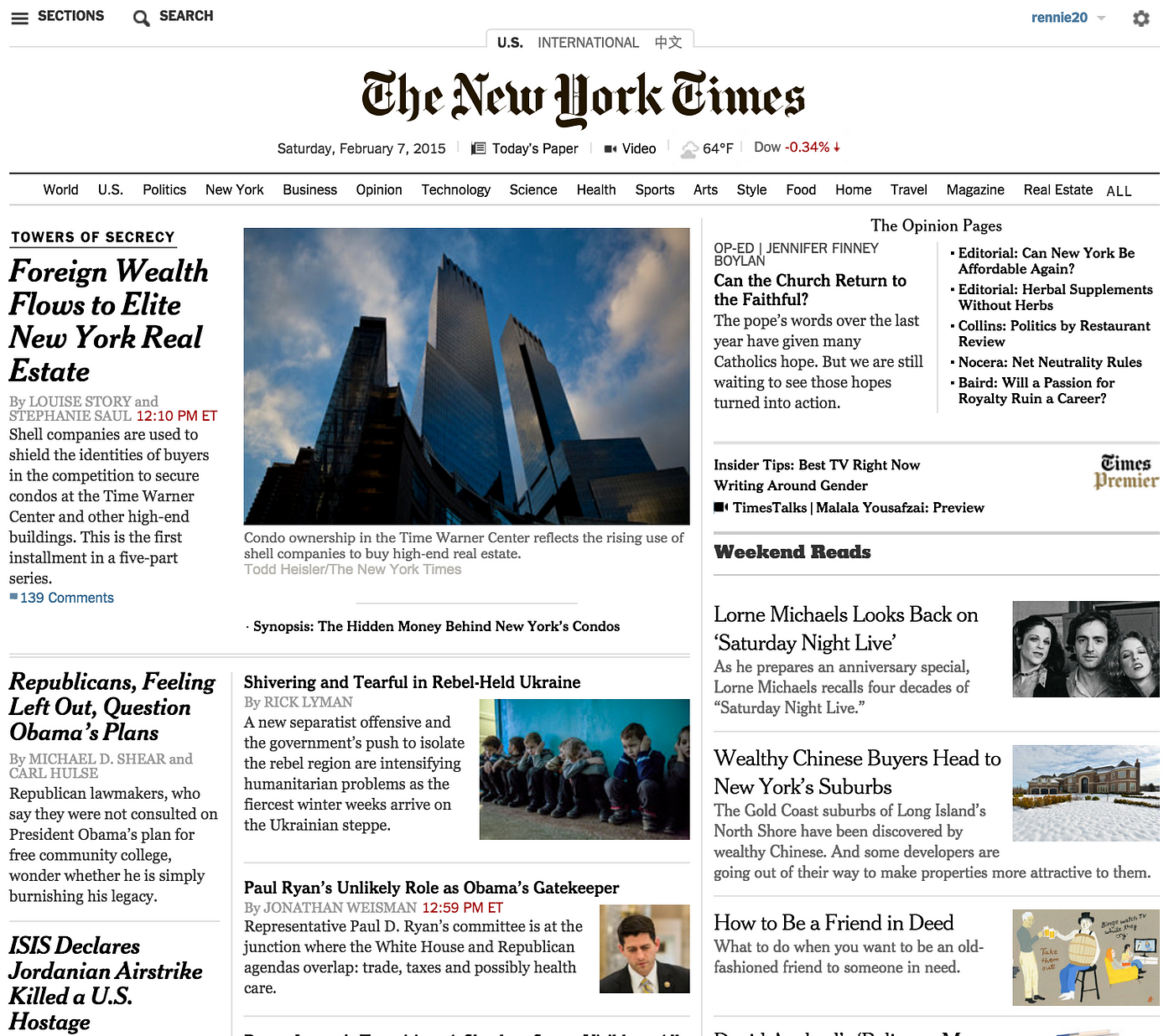The screenshot captured from the New York Times website features a clean, white background. In the upper left corner, there is a button for sections and a search button, while the upper right corner houses a settings gear icon and displays the username "Rennie20" in blue. Below this, the header reads "The New York Times, Saturday, February 7th, 2015," with the temperature noted as 64 degrees.

The front page is adorned with several images and headlines. Dominating the page is a photograph of condos at the Time Warner Center, accompanied by a caption highlighting the rising trend of using shell companies for purchasing high-end real estate. The associated article is titled "Towers of Secrecy: Foreign Wealth Flows to Elite New York Real Estate."

Other notable headlines include:
- "Republicans Feeling Left Out, Question Obama's Plans"
- "Shivering and Tearful in Rebel-Held Ukraine," illustrated with a poignant photo of small children crouched against a wall, holding their ears.
- "ISIS Declares Jordanian Airstrike Killed a U.S. Hostage"
- "Paul Ryan’s Unlikely Role as Obama’s Gatekeeper," featuring a photograph of Paul Ryan.
- "Weekend Reads: Lorne Michaels Looks Back on Saturday Night Live," paired with a black-and-white image of Lorne Michaels and Gilda Radner.
- "Wealthy Chinese Buyers Head to New York Suburbs," showcasing a large house.
- "How to Be a Friend Indeed," which includes a whimsical illustration of a man sitting on a stool wearing a barrel.